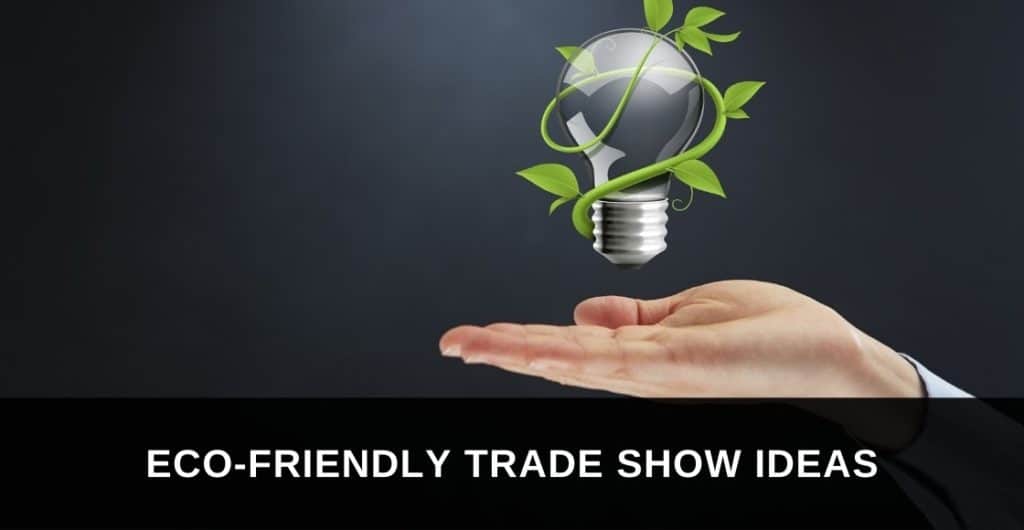This digitally generated poster features an advertising layout with a predominantly dark gray background that transitions to a slightly lighter shade towards the center of the image. At the bottom, a thick black horizontal bar spans from left to right, containing the white capitalized text "ECO-FRIENDLY TRADE SHOW IDEAS." Central to the composition is a floating, clear glass light bulb, subtly positioned a bit to the right of center. A green vine or branch with lush leaves intricately wraps around the bulb. Below this, a human hand with an open palm faces upwards, emerging from the lower part of the image, with a glimpse of the shirt sleeve visible. This striking visual symbolizes sustainability and innovation, ideal for conveying eco-friendly concepts.